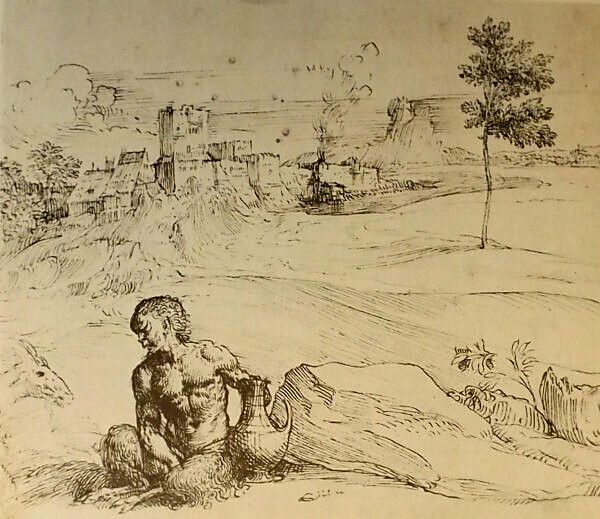This drawing appears to be a highly detailed and finely sketched illustration on faded, off-white parchment-like paper, either black and white or brown and white. The primary focus is a shirtless, kneeling male figure positioned in the bottom left corner. His legs are covered in shaggy fur, giving an impression of rugged wildness. He is holding a jug or urn with a handle and pedestal, and gazing to his right, where a goat's head can be seen peering in from the edge of the image. 

To the right of the man, there is a large rock and beyond it, some brush growing out of additional rocks. In the background, a solitary skinny tree rises towards the sky, beside a primitive cityscape with various buildings and trees. One of the structures has smoke trailing from its chimney, suggesting habitation. Further back, the horizon reveals a landscape with clouds and a distant mountain, possibly a volcano, all rendered with careful sketched details. The scene is marked by a high degree of shading and fine lines, creating a rich, evocative tableau that suggests both antiquity and intricate artistry.